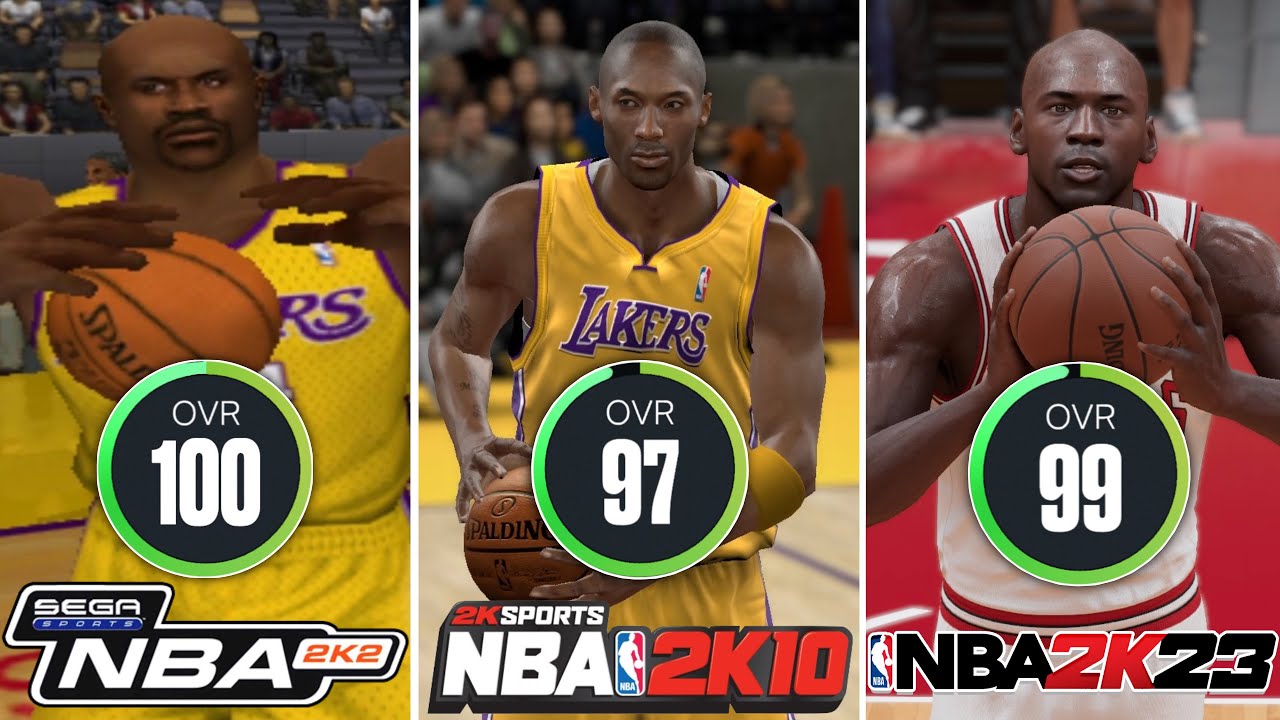The image displays three distinct basketball players each holding a basketball, highlighting the transition in quality and realism over different versions of a basketball video game series.

The first player, found in the leftmost image, is depicted in a poorly rendered, computer-generated visual. The proportions are noticeably off, with hands that appear incorrectly sized. The overall image is blurry, radiating low quality and artificiality. Centered within a green circle, the text "OVR100" is visibly marked, accompanied by "Siga NBA 2K2" beneath it.

Moving to the middle, the second image presents a considerable improvement in both clarity and detail. While it still retains a somewhat artificial appearance, possibly due to the player seeming cut-out and superimposed onto a blurred background, it approaches a more believable photographic quality. The player, donned in a yellow T-shirt, stands distinctly in focus against the defocused backdrop. In the center, a green circle displays "OVR97", and "2K Sports NBA 2K10" is inscribed below the image.

Lastly, the third player, showcased on the right, emanates the highest level of realism. Detailed features such as finger contours, muscle definition, and visible sweat illustrate a photorealistic portrayal. This player is clad in a red and white top. The green circle at the center reads "OVR99", with the text "NBA 2K23" appearing underneath.

Together, these images highlight the evolution of visual fidelity in the NBA 2K video game series over time.